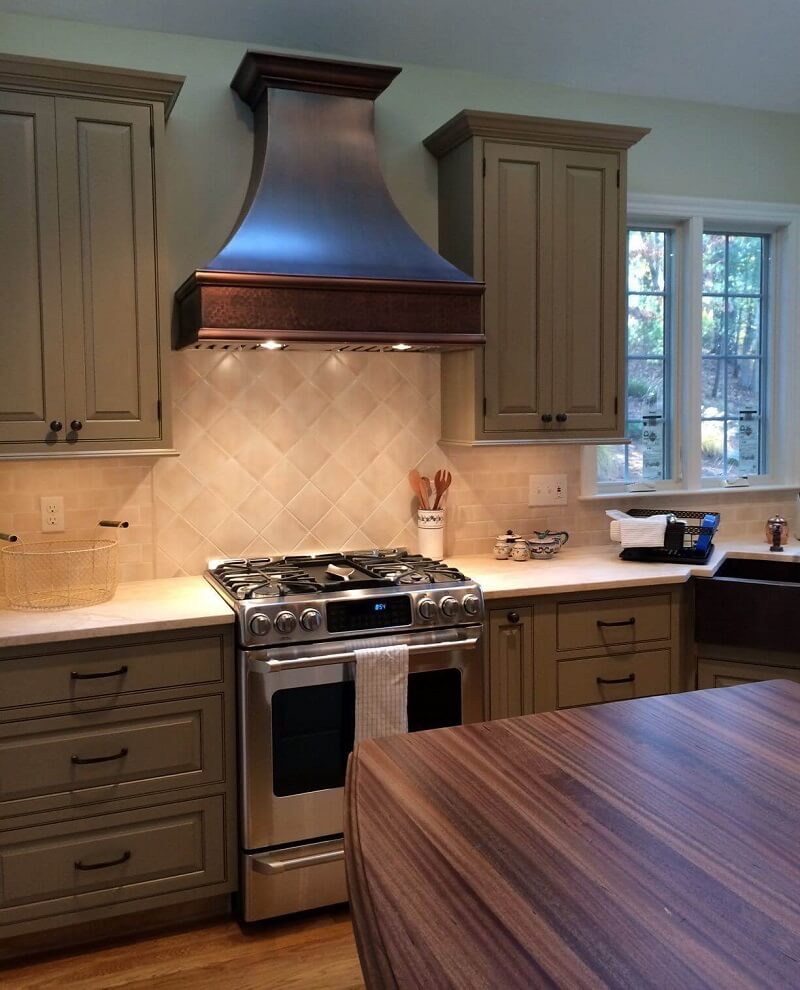The image showcases a neat and clean kitchen interior. In the foreground, a dark wooden countertop displays various accoutrements, including utensils like a wooden spatula, a glass ceramic teapot, salt and pepper, and other kitchen items. Moving into the background, light brown cabinets with small black handles are visible, paired with an olive green set of cabinets above and below the countertops. The centerpiece of the kitchen is a stainless steel stove with a tinted glass window, adorned with a white towel hanging from its handle. Above the stove, there is a copper-colored oven hood with two lights that illuminate the stainless steel stovetop and surrounding countertops. To the right of the cabinets, a window offers a daytime view of the outdoors, revealing a scene with trees and forestation, allowing natural light to enhance the ambiance. A basket sits on one of the counters, adding to the organized and tidy appearance of this modern kitchen space.